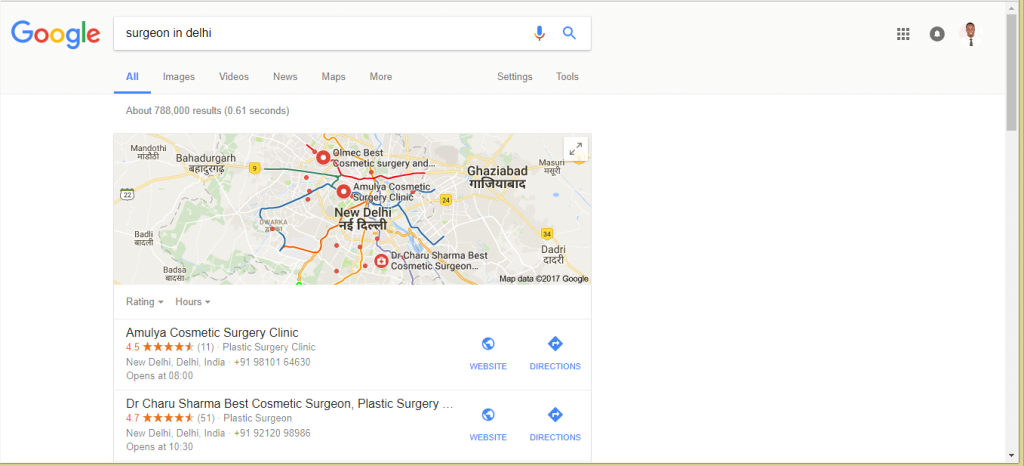The image is a screenshot of a Google search results page. At the top of the image, there's a grayish bar containing the Google logo in its signature blue, red, yellow, and green colors. Below the logo is a search bar with the query "Surgeon in Delhi." To the right of the search bar, there is a red, yellow, and blue microphone icon and a blue magnifying glass icon.

Beneath the search bar, several sub-menu options are listed: "All," highlighted in blue, followed by "Images," "Videos," "News," "Maps," "More," "Settings," and "Tools," all in gray. Below these options, the number of search results is displayed: approximately 788,000 results found in 0.61 seconds. 

At the top of the screen, you can also see some gray squares, a white and gray bell icon, and what appears to be a profile picture of a man in a suit.

Scattered beneath the search results count, there is a small Google Maps view featuring green, gray, red, and black color markers, with New Delhi positioned at the center of the map. The map also highlights various places of business with red markers and some gold number markings.

Below the map, search results offer sorting by rating and hours, indicated in gray text. 

The first result is the "Omula Cosmetic Surgery Clinic," rated 4.5 stars with 11 reviews, classified as a Plastic Surgery Clinic located in New Delhi, Delhi, India. The contact phone number is +91 9810164630 and it opens at 8:00 AM. There are two blue icons for the website (depicted with a globe) and directions (depicted with a diamond shape and an arrow).

The second result is "Dr. Charu Sharma, Best Cosmetic Surgeon," with a 4.7-star rating across 51 reviews. This clinic is also located in New Delhi, Delhi, India, with a phone number listed as +91 9212098986. It opens at 10:30 AM. Similar to the first result, there are blue icons for the website (globe icon) and directions (arrow icon).